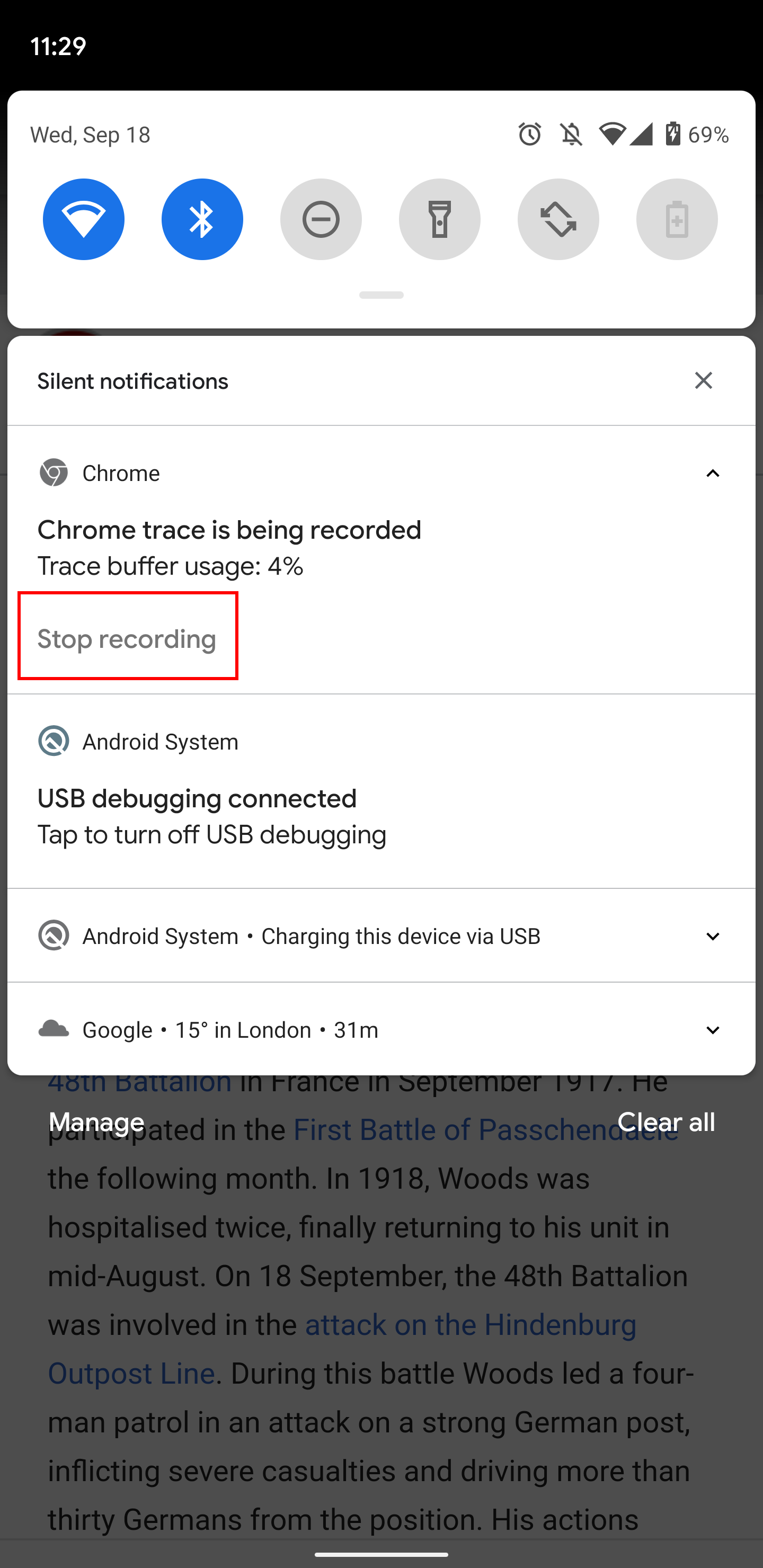A detailed caption for the image:

"This is a screenshot of a smartphone's notification and settings menu displayed on a mobile application screen with a black background. The top section features the date and status information, along with several icons. The Wi-Fi and Bluetooth icons are both blue, indicating they are active, while the 'Do Not Disturb' and flashlight icons are grayed out, implying they are inactive. A gray arrow icon, possibly for the Auto Rotate function, and the battery status are also visible. 

Below this, there is a section titled 'Silent Notifications' in black text, with an 'X' button on the far right to clear the notifications. The first silent notification is from Chrome, indicating that 'Chrome is being traced,' with the trace buffer usage at 4%. This notification has a red outline around a 'stop recording' option. Following this, there are two Android system notifications: one stating 'USB debugging connected' and another saying 'charging this device via USB.' The final piece of information at the bottom of the screen is the current temperature in London."